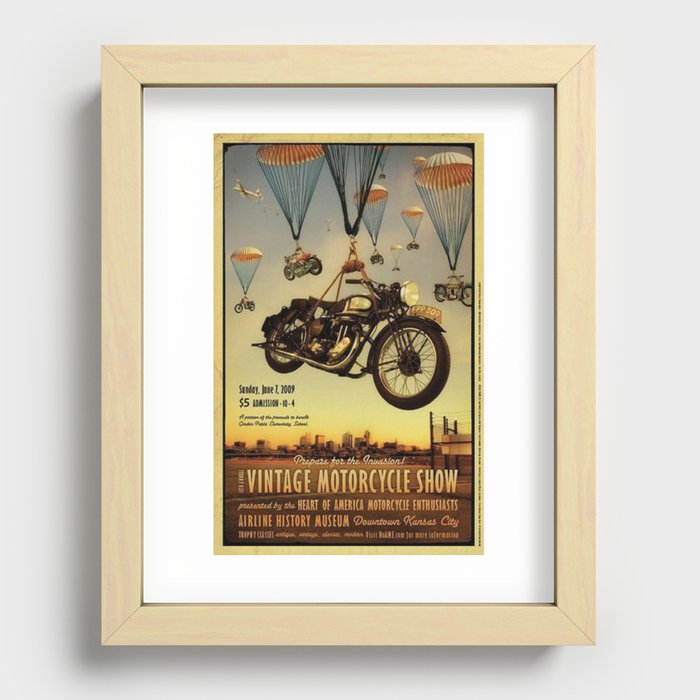The image depicts a flyer for a vintage motorcycle show, encased in a light brown, unfinished wooden frame hanging on a white wall. Inside the frame, the flyer features a detailed illustration of several motorcycles parachuting down to the ground, accompanied by hot air balloons and a large white plane in the top left corner. Prominently displayed in black text towards the middle left of the flyer are the event details: "Sunday, June 7, 2009. $5 admission, 10 to 4." At the bottom, the flyer bears the headline, "Prepare for the Invasion," and states, "Vintage motorcycle show presented by the Heart of America Motorcycle Enthusiasts," held at the Airline History Museum in downtown Kansas City. The bottom section contains some additional text that is blurred and difficult to read.